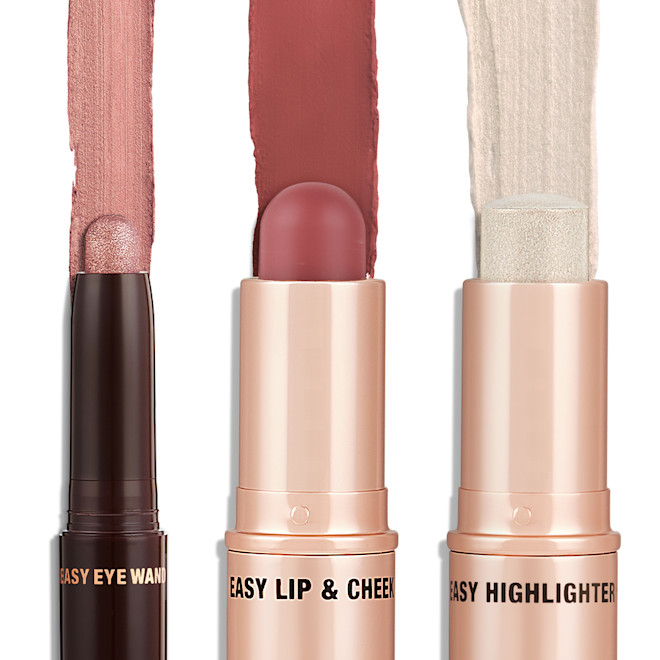The photograph features three distinct makeup products aligned from left to right against a solid white background, each demonstrating its unique color and finish with visible streaks. The product on the left is a black tube with a round metallic pink bulb protruding from the top, emitting a pink glittery streak. This tube is labeled "Easy Eye Wand" in gold text, suggesting it's an eye makeup product. The middle product is a slightly thicker, champagne-colored tube adorned with black text that reads "Easy Lip and Cheek." It reveals a dark brick red bulb, with a corresponding streak extending upward. The rightmost product mirrors the middle in tube color and size, also featuring black text that reads "Easy Highlighter." It showcases a glimmering iridescent white bulb with a sparkling white streak trailing along the white background.